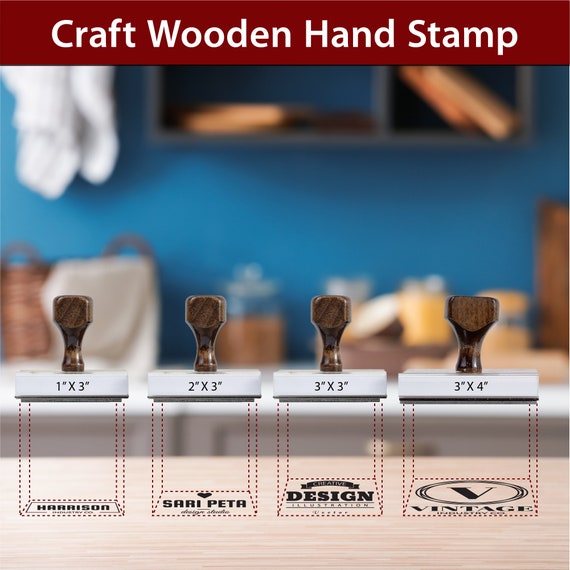The image depicts a set of craft wooden handle stamps prominently displayed against a blurred background of a blue-walled room with floating shelves, baskets, and jars on the floor. At the top of the image, in white text enclosed by a dark red, almost black, rectangular border, it reads "Craft Wooden Hand Stamp." Below this header, four wooden handle stamps are neatly arranged in a row on a light-colored wooden platform, each showcasing a different size and label. The stamps, with their glossy, dark walnut-colored wooden handles and white bases, are standing upright as if ready to be stamped. They are labeled from left to right as follows: the first stamp, measuring 1 inch by 3 inches, is marked "Harrison"; the second, 2 inches by 3 inches, says "Sorry Peter"; the third, 3 inches by 3 inches, reads "Design Illustration"; and the fourth, 3 inches by 4 inches, is labeled "Vintage" with a prominent letter 'V'. Dotted red lines extend downward from each stamp, illustrating the dimensions of the impression they would make. The overall setup blends a tidy, detailed focus on the stamps with a softly blurred, homely atmosphere in the background.